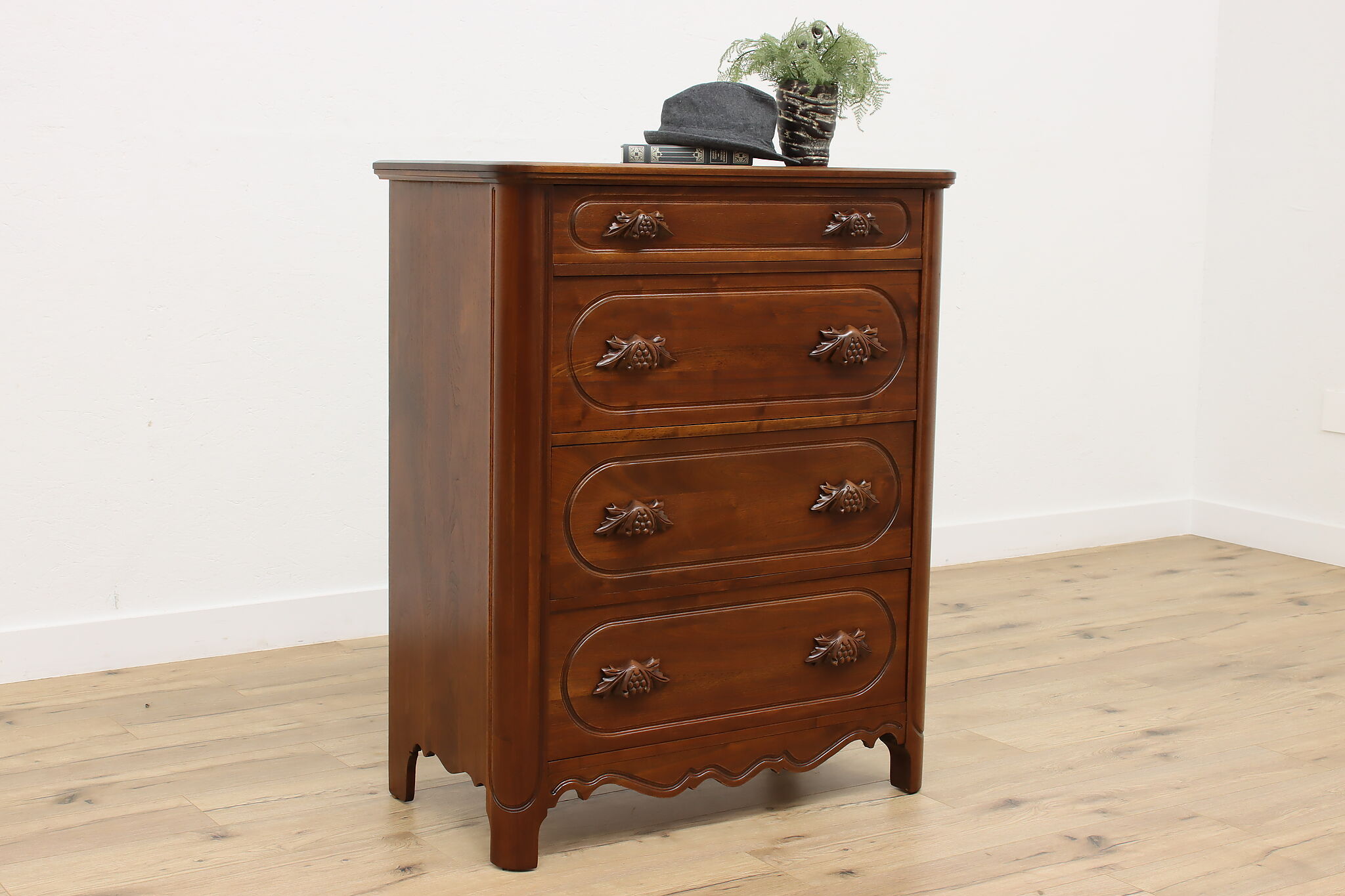This color photograph captures a simple, clean corner of a room featuring a meticulous, light cherry wooden chest of drawers. The room has stark white walls with no decorations, complemented by natural oak-paneled hardwood flooring. The chest stands out in the center with its four drawers, adorned by Germanic, forest-inspired carved wooden pulls. On top of the dresser are a few carefully arranged items: a small, handmade clay vase containing wispy green fern fronds, a book, and a gray man's hat resting atop the book. The dresser, in excellent condition, presents oval designs on its rectangular drawer fronts, enhancing its straightforward yet elegant aesthetics.